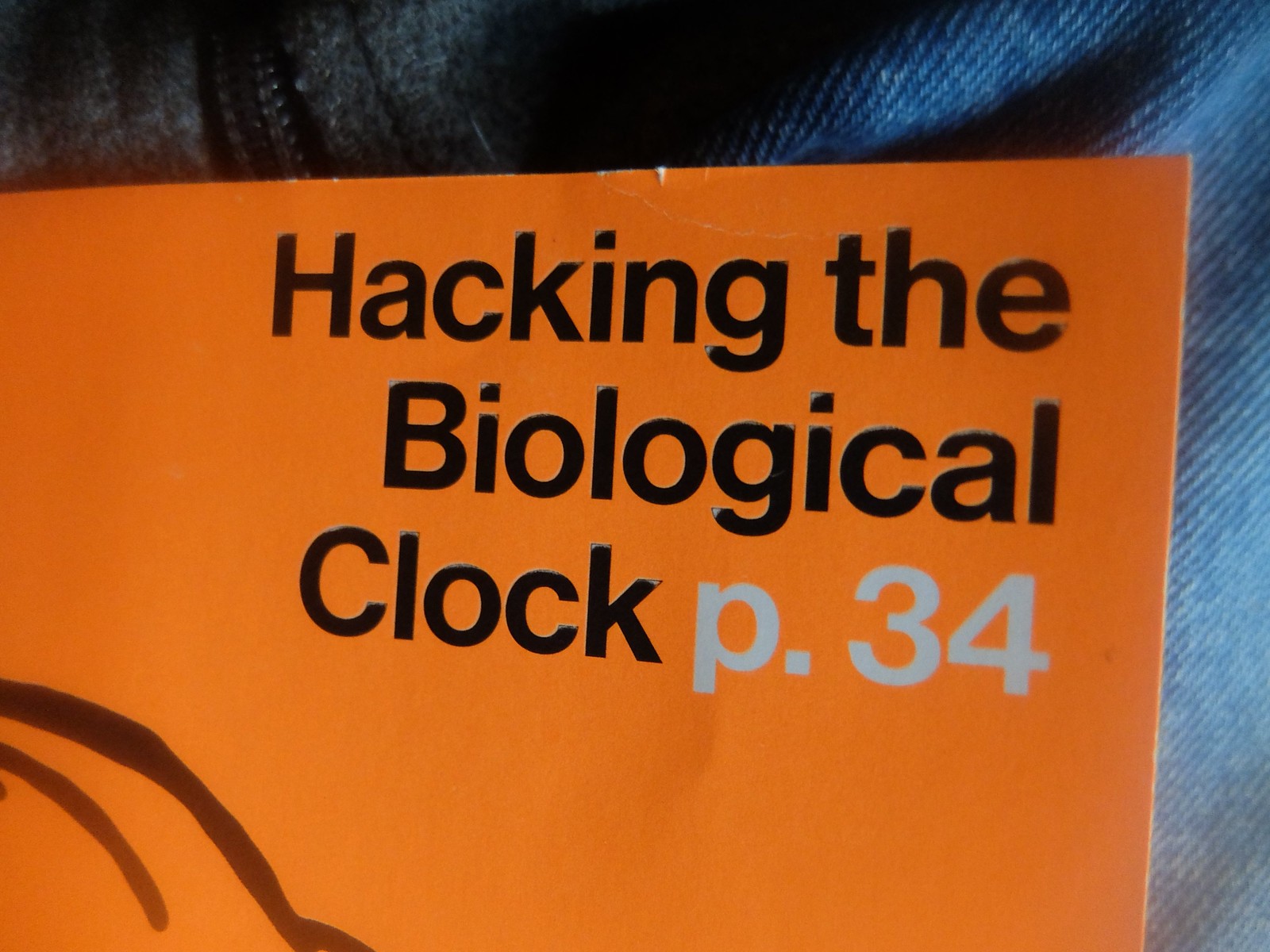The image depicts a slightly worn orange book titled "Hacking the Biological Clock" in bold black letters. The cover also indicates "page 34" in smaller, gray letters. The book lies atop a pair of jeans, evident from the thick, textured material surrounding it. The jeans feature a zipper, suggesting the presence of a jacket or similar garment. Diagonal lines cross the book's cover from the left side, adding a decorative element to the image.